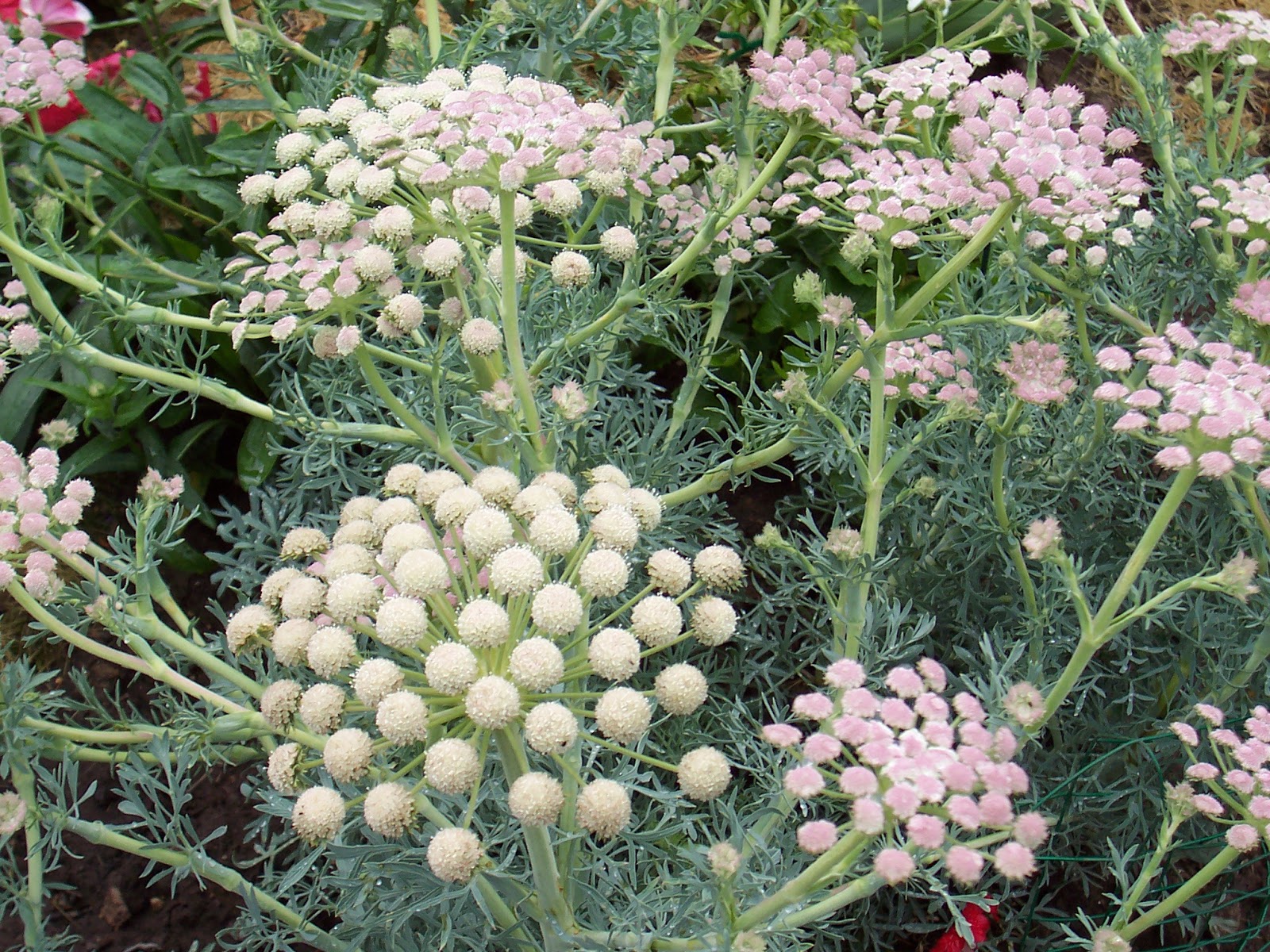The photograph captures a vibrant section of a flower patch, possibly from a backyard garden or botanical space. Prominently featured are unique flowering plants with distinct, round inflorescences that bear a resemblance to small cotton balls or delicate snowballs. These blooms, appearing in off-white, pink, and hints of purple, emerge from thick green stalks amongst a dense backdrop of green foliage. The flowers consist of clusters of tiny round blossoms that protrude from a central stem, with each cluster branching out, much like the structure of broccoli. Below these flowering heads are finer, darker leaves, adding depth to the lush landscape. Subtle hints of red among the blooms suggest other floral varieties interspersed within the garden, adding a pop of contrasting color. The overall composition is a harmonious blend of green stems, intricate leaves, and bursts of white and pink flower heads, creating a truly captivating and richly detailed scene.